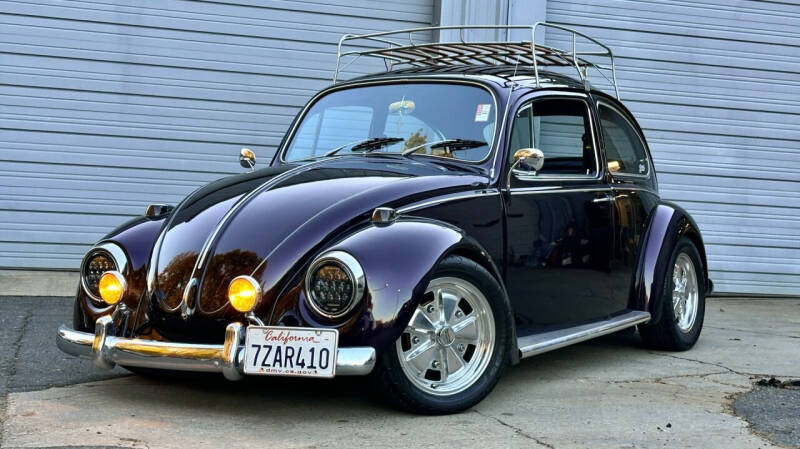This image features a meticulously maintained vintage Volkswagen Beetle, likely from the 1950s or 60s. The car boasts a striking deep purple-blue paint job which shines brilliantly. Notably, it has yellow main headlights, smaller secondary headlights, and chrome or silver accents including rearview mirrors, running boards, and wheels. The front bumper and headlamp housings are also chromed, contributing to a cohesive, polished appearance.

A silver metal roof rack, suitable for carrying luggage or other materials, is mounted atop the car. The car features a California license plate with the registration number 7ZAR410. Through the open front window, a yellow rear-view mirror and a windshield sticker are visible.

The Beetle is parked on a somewhat worn concrete area that appears to have been patched with asphalt. This is situated in front of a double garage with blue-gray, slatted doors that give off a warehouse vibe. Overall, the car exudes a snazzy look, standing out against the more rugged backdrop.